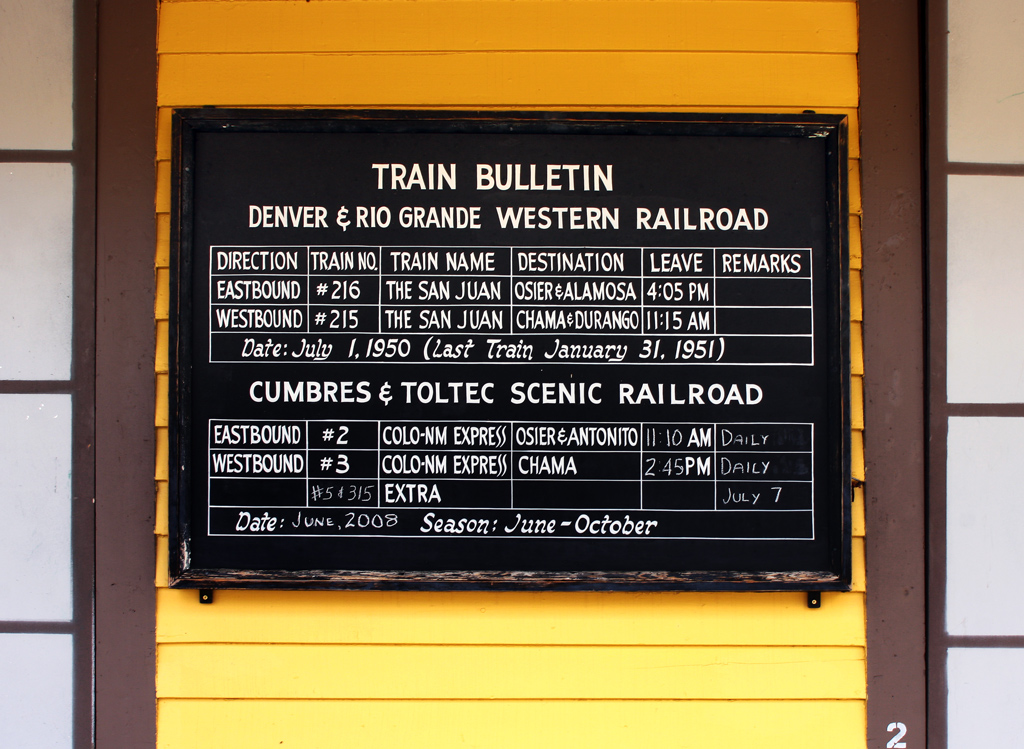The image features a historic black train bulletin sign with white text, fixed to a yellow background resembling shutters, framed in dark brown, against a wall with white tiles. The sign prominently displays "Train Bulletin" at the top, followed by "Denver and Rio Grande Western Railroad." Below this, there is a detailed grid outlining train schedules with columns labeled Direction, Train Number, Train Name, Destination, Leave, and Remarks. The entries include eastbound and westbound directions with train numbers 216 and 215 respectively, both named "The San Juan". The destinations listed are Oseer and Alamosa for eastbound, and Chama and Durango for westbound. Additionally, the sign notes historical dates including July 1, 1950, and January 31, 1951. Below these details, there is another section for the Cumbres and Toltec Scenic Railroad, marking further schedules and a season running from June to October, 2008.